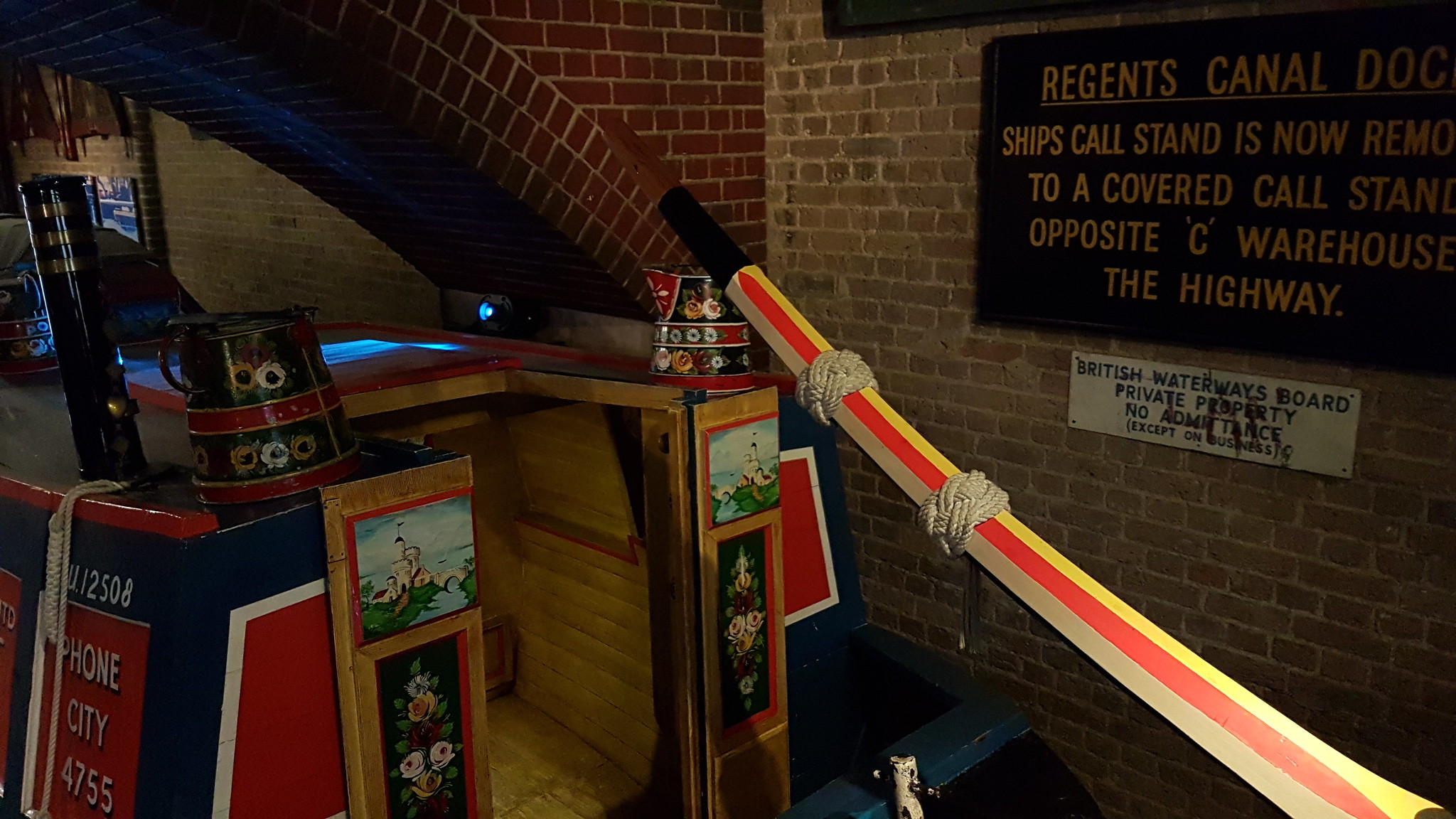The image depicts the interior of what appears to be a bar or a potentially themed museum exhibit. Central to the scene is a staircase leading down into the space, with a prominent guardrail that is colored brown, red, and yellow. At the bottom of the stairs, there is a counter or bar area, with various pictures displayed on it. To the right of the counter, a brick wall—tan and red in hue—displays several signs. One sign reads, "Regions Canal," another partially visible sign mentions, "Ship's call stand is now remote to a covered call stand opposite Sea Warehouse, the highway." Other signs include, "British Waterways Board, private property, no admittance except on business," and "Phone City 4755," with a mixture of colors including black, white, yellow, and blue. 

To the left of the guardrail, there’s a wooden cart with two buckets on either side and painted decorations that include houses and flowers. Along the walls are objects such as some ropes and more bricks extending into the background, adding texture to the scene. The overall setting evokes a lower-level bar with vintage decorations and signs, contributing to a rustic, historical ambiance.